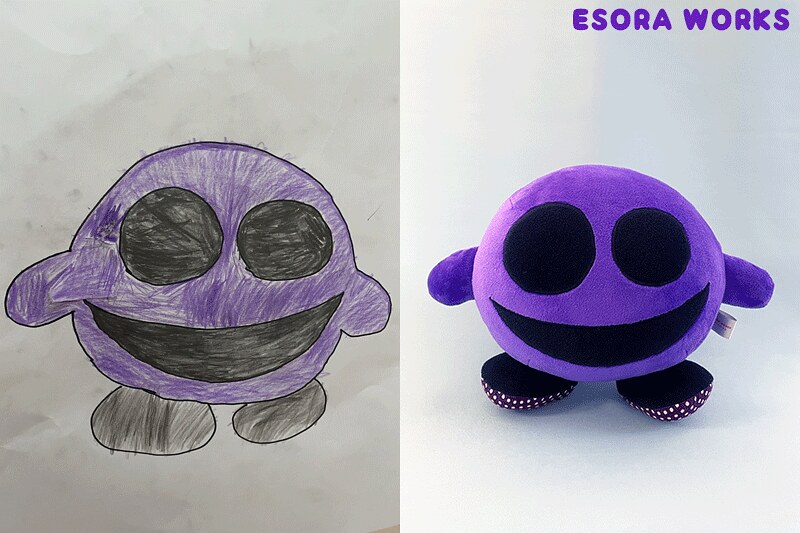This photograph features a creative split design. On the left side, there is a child's drawing rendered on a white piece of paper, which shows a lovable monster with a purple crayon body and head. The monster has big black eyes, a black mouth, and round black feet. The paper appears slightly folded, adding an authentic touch.

On the right side of the photograph, we see a plush toy replica of the same creature, created by a company named Esora Works (as indicated by the text at the top of the image). The plush monster faithfully mirrors the drawing, showcasing a spherical purple body with two purple arms sticking out from its sides. It also has a small white label attached to it. The plush version maintains the original design’s black eyes, black mouth, and round black feet, with additional purple and white dots underneath the feet, adding a whimsical touch.